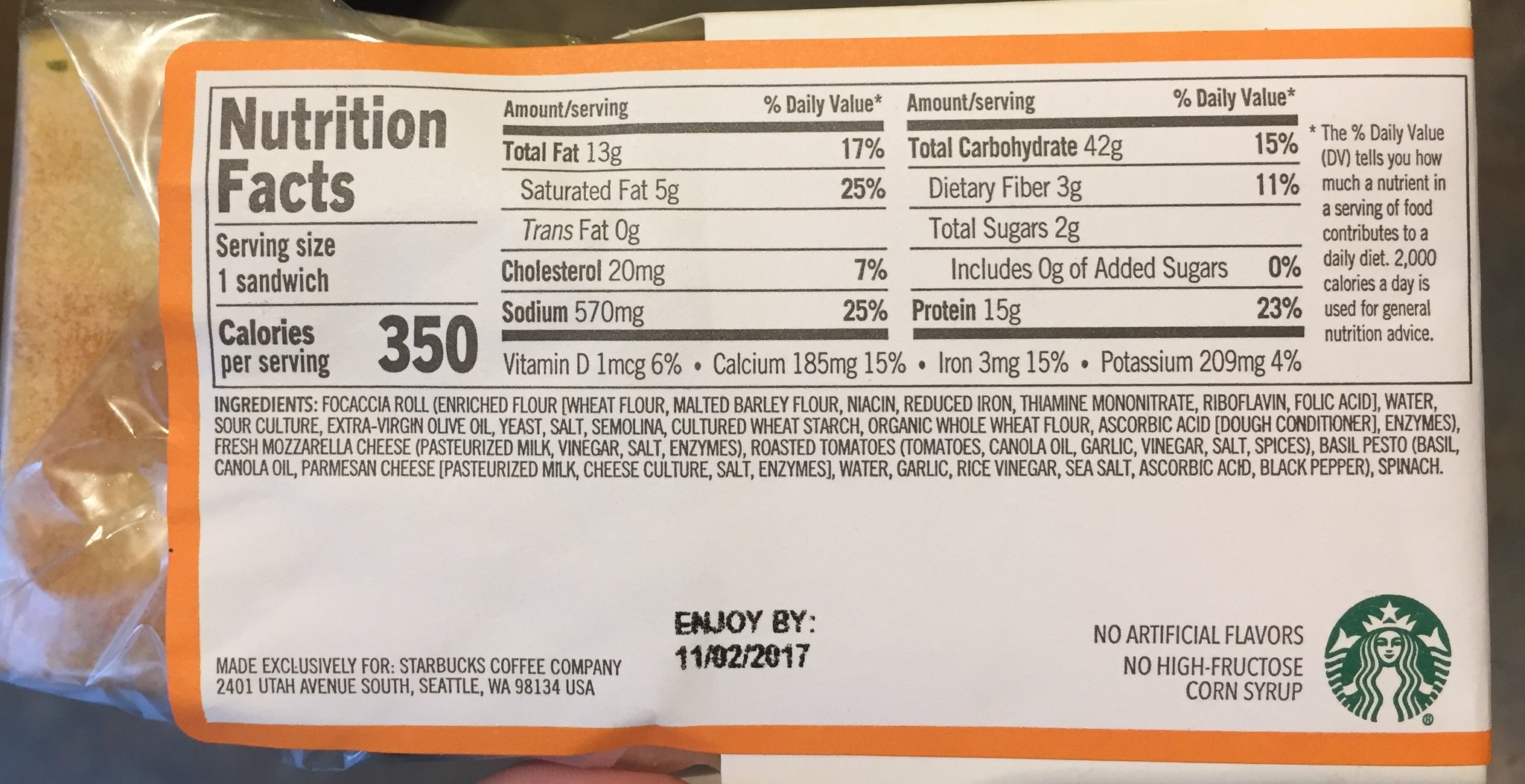This photograph showcases the back of a packaged sandwich encased in clear plastic. Prominently displayed on the packaging are detailed nutrition facts. The serving size clearly states "one sandwich," with each serving containing 350 calories. Adjacent to this, a comprehensive list of nutritional information in black text includes the total fat, saturated fat, cholesterol, sodium, total carbohydrates, and total sugars.

Below the nutrition facts, we find a list of ingredients, also written in black. The ingredients include bread, salt, vinegar, enzymes, various cheeses, extra virgin olive oil, tomatoes, and garlic. Further down, the "enjoy by" date is indicated as 11-02-2017.

On the right side of the packaging, the iconic Starbucks logo is visible. The logo features a white mermaid with a dark green background. Nearby, in black text, are affirmations of the product's quality, stating "no artificial flavors" and "no high fructose corn syrup." The nutrition facts label is emphasized by a bright orange border, making it stand out against the clear plastic of the sandwich packaging.